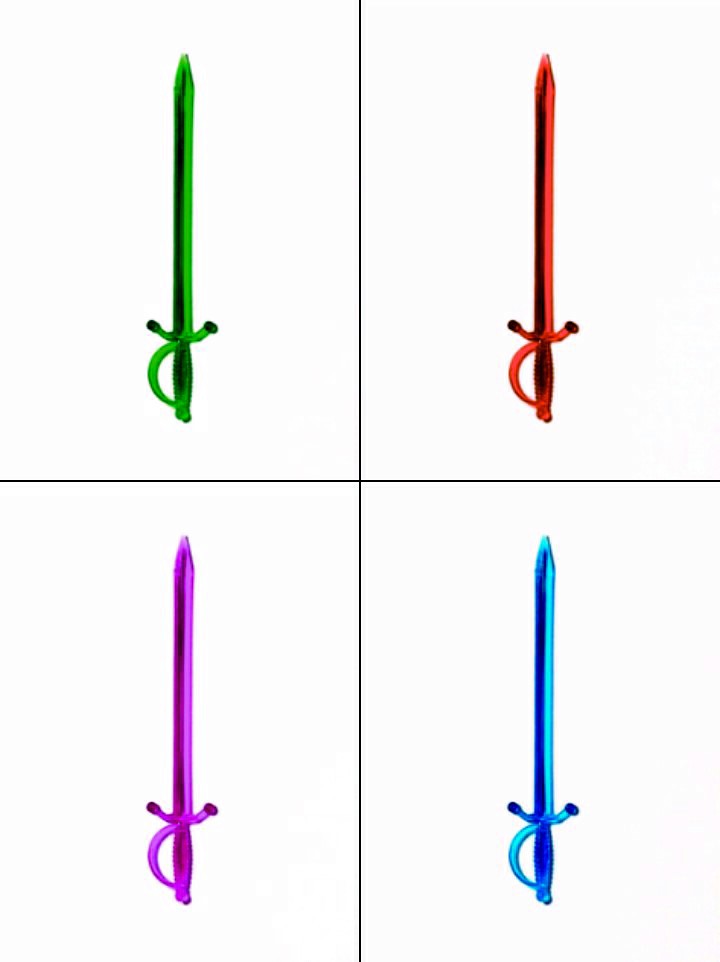The image is a rectangular graphic divided into four quadrants by a black vertical line intersecting a black horizontal line at the center. Each quadrant contains an identical sword, distinguished only by color. The sword in the top left quadrant is shaded in bright green with darker green shadows. In the top right quadrant, the sword is rendered in red with darker red shading. The bottom left features a sword in fuchsia magenta purple, including complementary darker tones. The sword in the bottom right quadrant is medium blue with darker blue accents. All swords have a metallic appearance with a nearly circular handle, positioned vertically with blades pointing upward. The background is plain white, accentuating the simple yet striking design of the swords, which could resemble metallic knitting needles due to their pointed tips and reflective quality.